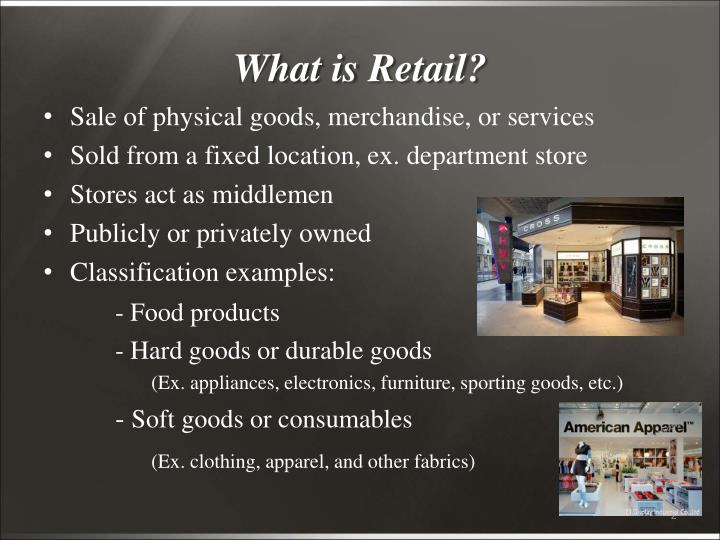The image is a gray PowerPoint slide with a slightly lighter gray in the upper right and slightly darker gray in the lower left. In the upper left corner, a diagonal light-colored line breaks the monochrome background. The slide is titled in the middle at the top with the white text, "What is retail?" Below the title, five primary bullet points in white font read: "Sale of physical goods, merchandise, or services," "Sold from a fixed location (e.g., department store)," "Stores act as middlemen," "Publicly or privately owned," and "Classification examples." This last point is followed by three sub-bullet points: "Food products," "Hard goods or durable goods (e.g., appliances, electronics, furniture, sporting goods, etc.)," and "Soft goods or consumables (e.g., clothing, apparel, and other fabrics)."

On the right-hand side of the slide, there are two photographs. The first, centered in the middle right, depicts the exterior of a store in a mall, potentially a watch or pen store, with the word "Cross" visible on its sign. Below this, in the bottom right corner, is a picture of an American Apparel store, showing a mannequin in an outfit and various clothes stacked on tables.